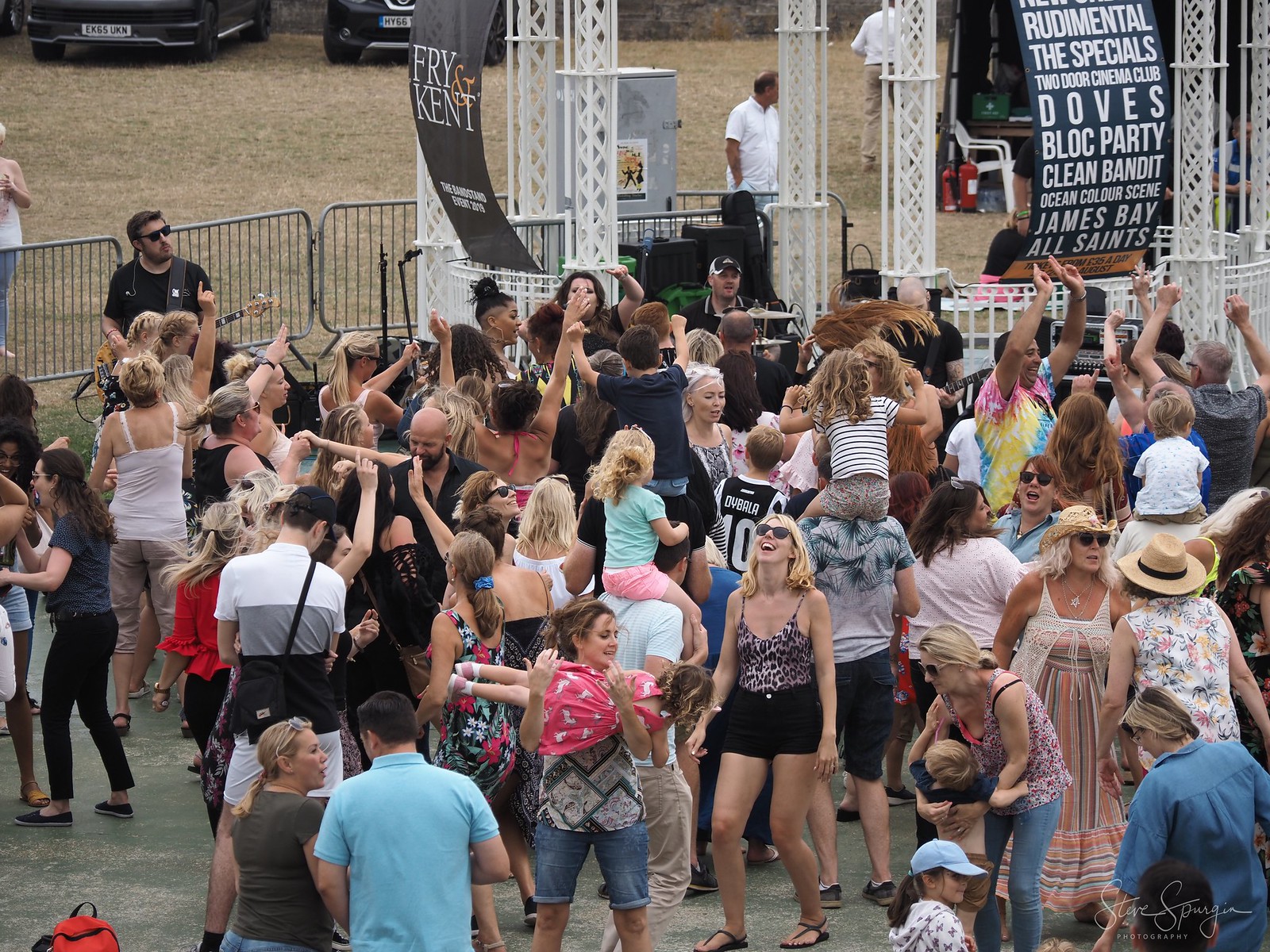The image depicts a vibrant outdoor music festival during the daytime, featuring an exuberant crowd of people enjoying the live performances. The scene is set on a hard concrete surface with a stage in the background adorned with banners listing band names such as Fry and Kent, Rudimental, The Specials, Two Door Cinema Club, Doves, Block Party, Clean Bandit, Ocean Color Scene, James Bay, and All Saints. The crowd, dressed in summery attire including sundresses, tank tops, and shorts, is a mix of adults and children, indicating a family-friendly atmosphere. In the foreground, numerous attendees are dancing and milling about. Despite the overcast sky, the atmosphere is festive and lively. Musicians including a guitarist, a drummer, a female singer, and a male bass player are barely visible behind the enthusiastic audience. Additional elements include parked cars and grass visible in the upper left-hand corner, separated from the gathering by temporary metal barriers. This photograph, signed by Steve Spurgeon Photography, captures the joyous essence of a communal musical experience.